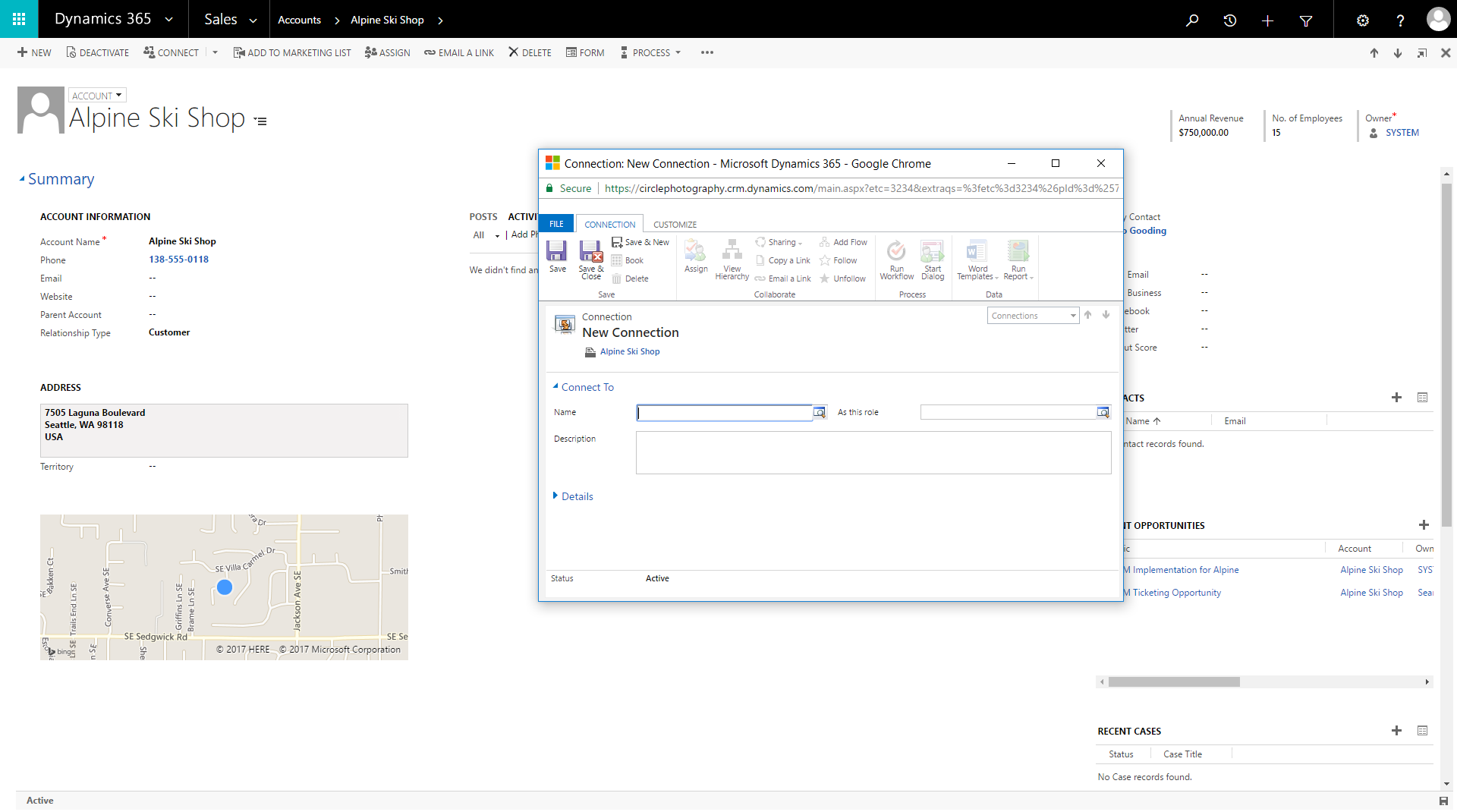This screenshot from a Dynamics 365 webpage, viewed in Google Chrome, features a centrally positioned pop-up window titled "Connection: New Connection." Below the title, a web address is visible. The pop-up window includes a navigation menu and several actionable buttons, such as "Save" and "Save and Close." The primary content of the pop-up is divided into sections: the "Connect To" section with input boxes for "Name" and "Description," and the "Details" section, which is collapsible, indicated by a blue expandable arrow next to the text "Details."